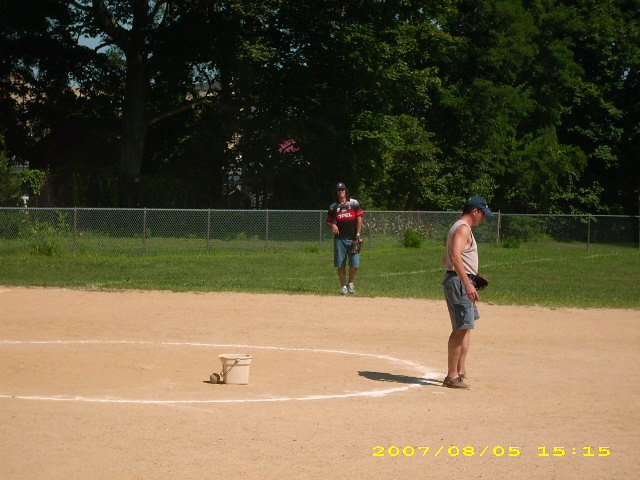The dated image, taken on August 5th, 2007, at 3:15 PM, captures a scene at a baseball field with a clear, somewhat vintage quality. In the foreground, two men in shorts are positioned on a dirt area surrounded by a lush green grassy field. The man on the left wears a dark hat, a black shirt with white shoulders and red accents, jean shorts, and white shoes, while the shirt on his back displays the word "OPEL" in white text inside a red square. He stands near the edge of a white chalk circle. The other man, wearing a blue hat, a light-colored tank top, gray shorts, and brown shoes, stands directly in front of the circle with a baseball mitt clenched in his hand. In the middle of this chalk circle is a bucket, with a baseball lying beside it. Behind the dirt pitcher's mound, a chain-link fence and a line of trees frame the serene backdrop.